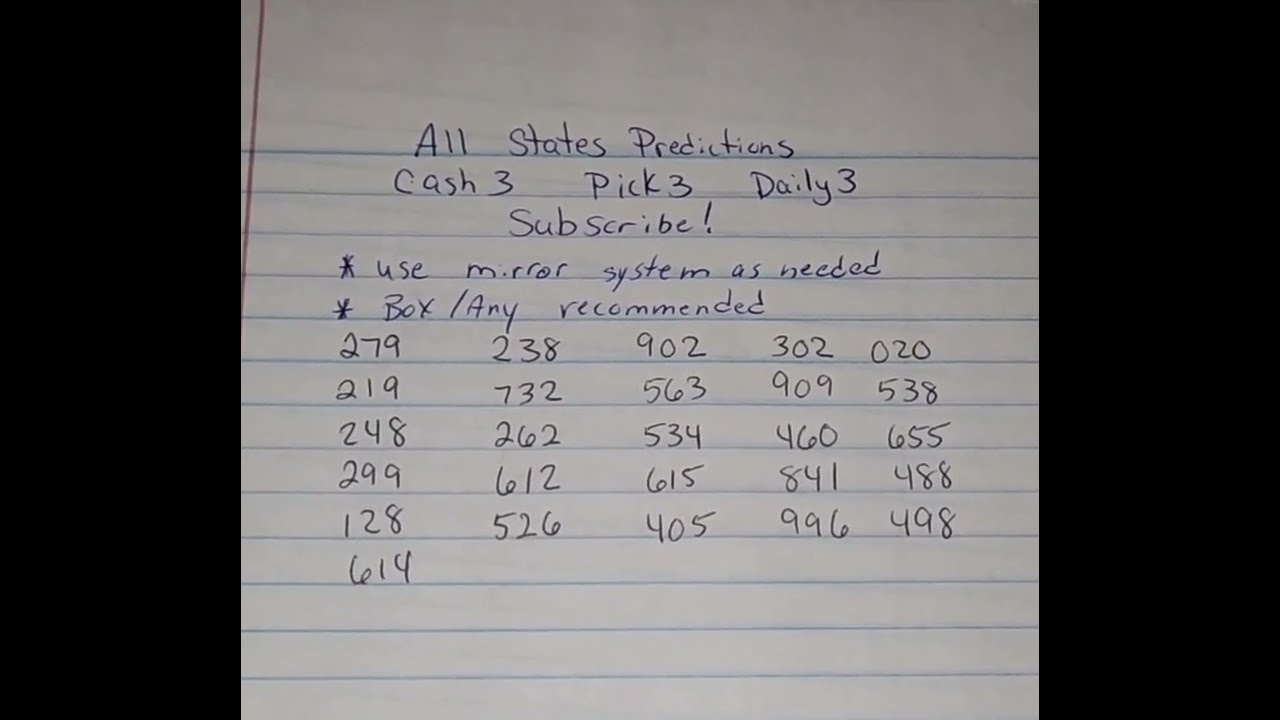The photorealistic image depicts a piece of white or grayish notebook paper with blue horizontal lines and a red vertical margin on the left. Written in blue pen at the top of the page is the title "All States Predictions," under which are the words "Cash 3, Pick 3, Daily 3." Below this, the word "SUBSCRIBE!" is prominently written with an exclamation mark. Further down, there are two bullet points, each marked with a star: the first reads "Use Mirror System as Needed" and the second "Box/Any Recommended." Beneath these instructions, five columns of numbers are listed in vertical alignment. The first column contains the numbers 279, 219, 248, 299, 128, and 614. The second column includes 238, 732, 262, 612, and 526. The third column lists 902, 563, 534, 615, and 405. The fourth column has the numbers 302, 909, 460, 841, and 996. The fifth and final column consists of 020, 538, 655, 488, and 498.